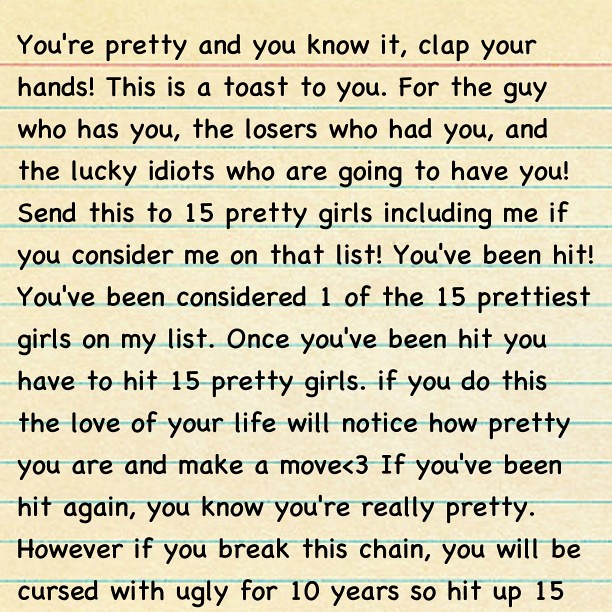The image displays a piece of wide-lined, yellow notebook paper with turquoise lines and a red top line. The text, written in black pre-printed font, reads: 

"You're pretty and you know it. Clap your hands! This is a toast to you: for the guy who has you, the losers who had you, and the lucky idiots who are going to have you! Send this to 15 pretty girls, including me if you consider me on that list! You've been hit! You've been considered one of the 15 prettiest girls on my list. Once you've been hit, you have to hit 15 pretty girls. If you do this, the love of your life will notice how pretty you are and make a move <3. If you've been hit again, you know you're really pretty. However, if you break this chain, you will be cursed with ugly for 10 years. So hit up 15."

This image is an example of a chain letter commonly circulated among adolescent girls.